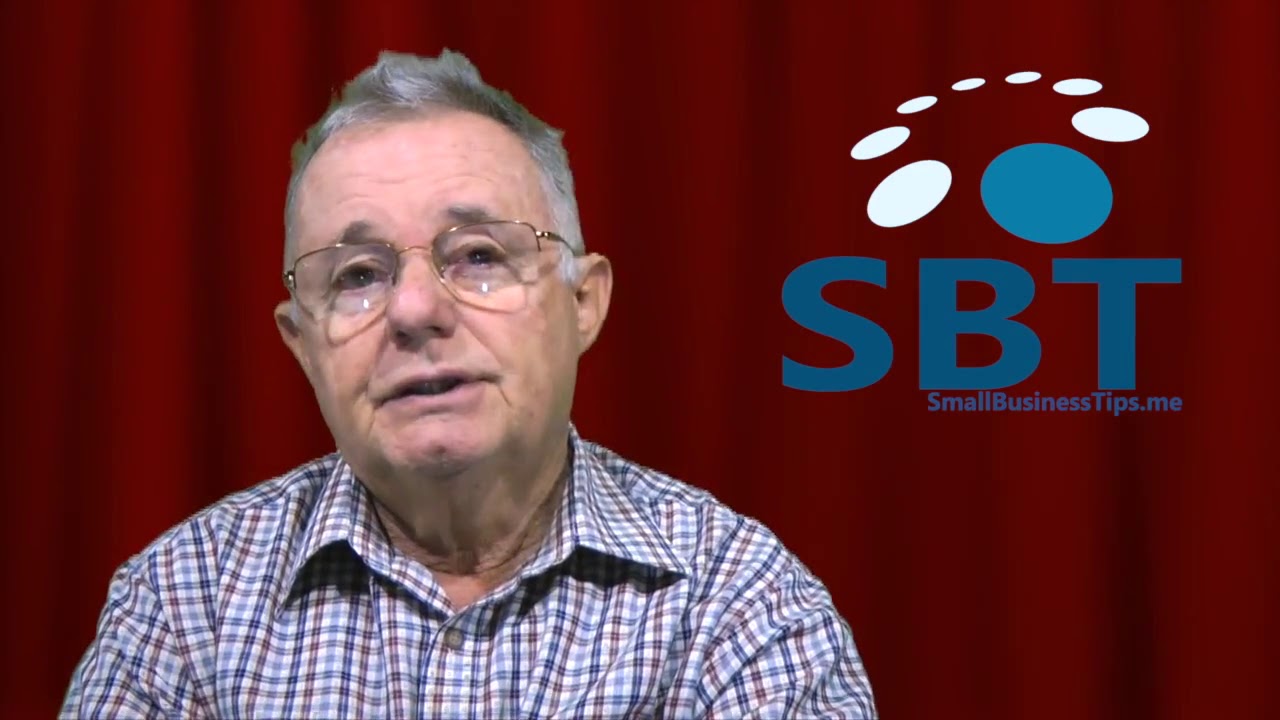The image appears to be a screenshot or an advertisement featuring an older gentleman in his 60s, situated in front of a semi-blurred, dark red theater curtain. The man, who is standing slightly to the left, has short gray and silver hair, wears wire-frame glasses, and has dark eyebrows. He is dressed in a long-sleeve, button-down plaid shirt that features shades of white, blue, and brown. His expression is serious, and his mouth is slightly open, as if he is about to speak. To the right of the man, there is a prominent logo with a large blue circle and an arc of white circles above it. Below the logo, the text "SBT" is written in bold blue capital letters, and underneath, the website "smallbusinesstips.me" is displayed in smaller blue font.